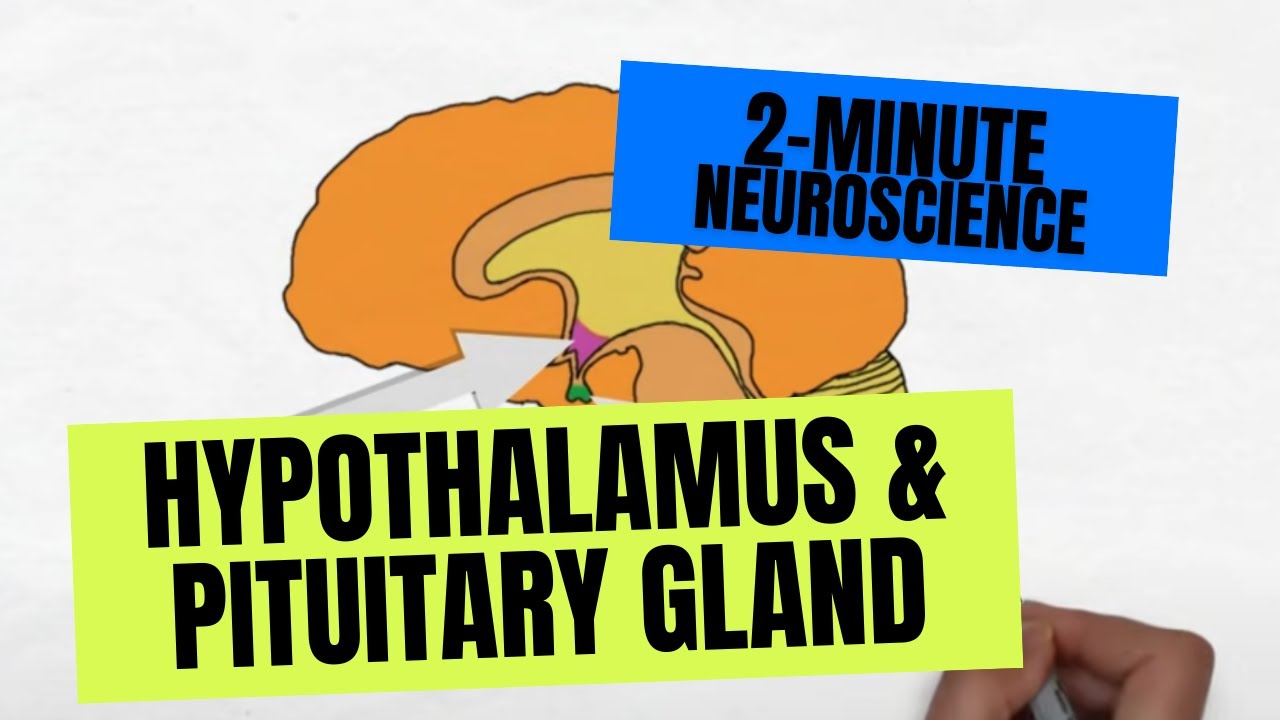The image features a colorful illustration of a brain at its center, with dominant hues including yellow in the middle and shades of peach, tan, and orange surrounding it. Overlapping the brain is a blue rectangle at the top that reads "Two-Minute Neuroscience" in black letters. Below this, a larger yellow rectangle displays the title, "Hypothalamus and Pituitary Gland," also in black letters. An arrow, white in color, extends from this yellow rectangle pointing towards the hypothalamus and pituitary gland area of the brain, which is depicted in pink. In the lower part of the image, partially obscured by the yellow rectangle, a person's right hand is visible, holding a pen, adding an element as if they are actively drawing or highlighting parts of the brain. This suggests the image might be from a presentation or an educational video.